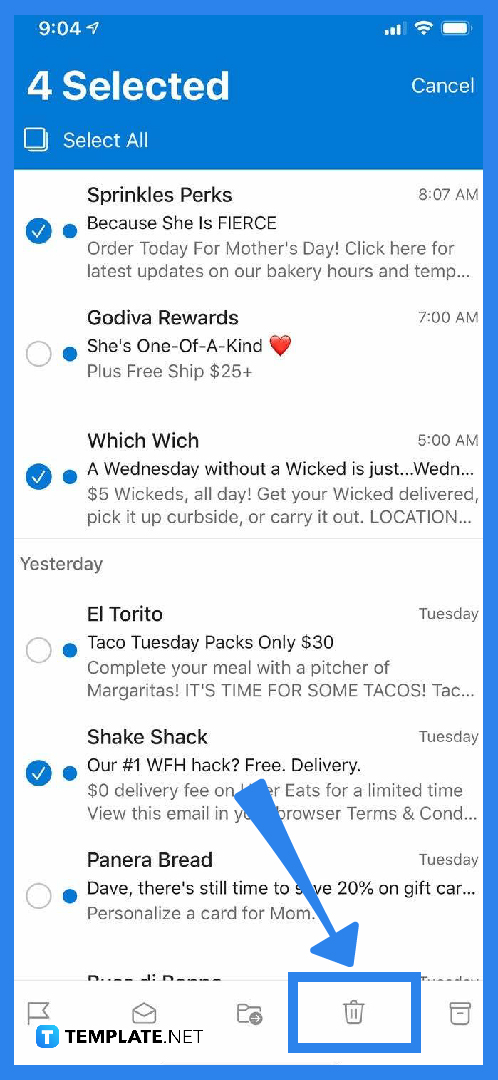In this screenshot taken from a cell phone, you can see the status bar at the top left corner displaying "9:04" with a small arrow next to it, along with icons for signal bars, Wi-Fi, and battery status. These elements are all rendered in a dark royal blue color. The entire screen has a border in a lighter shade of royal blue, creating an inset box effect.

At the top of the screen, in white text, you see "Selected" on the left side and "Cancel" on the right side. Below the "Selected" label is another option that says "Select All." The main content area features a white box with various items listed as if in an email inbox. Each list item is written in white text against a blue background, indicating selected items.

One prominently selected item is a promotion, highlighted in solid blue with a blue checkmark dot, stating, "Order Today for Mother's Day" at 8:07 AM. Following this promotional item are other list entries including "Godiva Rewards" and "Which Which, a Wednesday without a Wicked." Additionally, there is a noteworthy circle indicating a checked item and a giant blue arrow pointing towards a "Trash" button, emphasizing the option to discard messages.